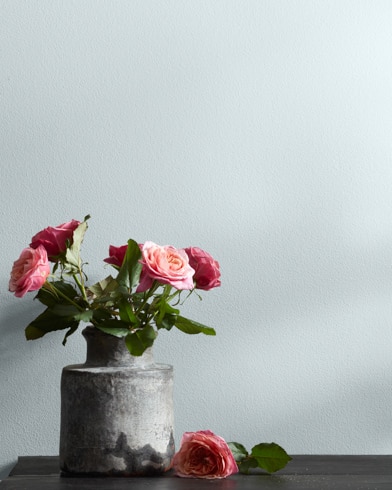In the photograph, a peculiar vase commands attention with its unusual, T-shaped design. The vase, seemingly crafted in an amateur pottery class, is marked by rough textures and lopsided, abrupt transitions from its wide cylindrical base to a narrower top. Its dark and light gray hues are accented by darker spots, adding to its unpolished appearance. The vessel houses five healthy, pinkish-red roses with vibrant leaves, and one rose of matching color lies on a dark wooden table with a ledge that attaches to the surrounding wall. The backdrop is a consistent light gray, placing the focus squarely on the contrast between the aesthetically pleasing, well-watered roses and the rough, ungainly vase they inhabit. The entire arrangement is situated to the left side of the image, which is cropped tightly, cutting off a portion of the table.